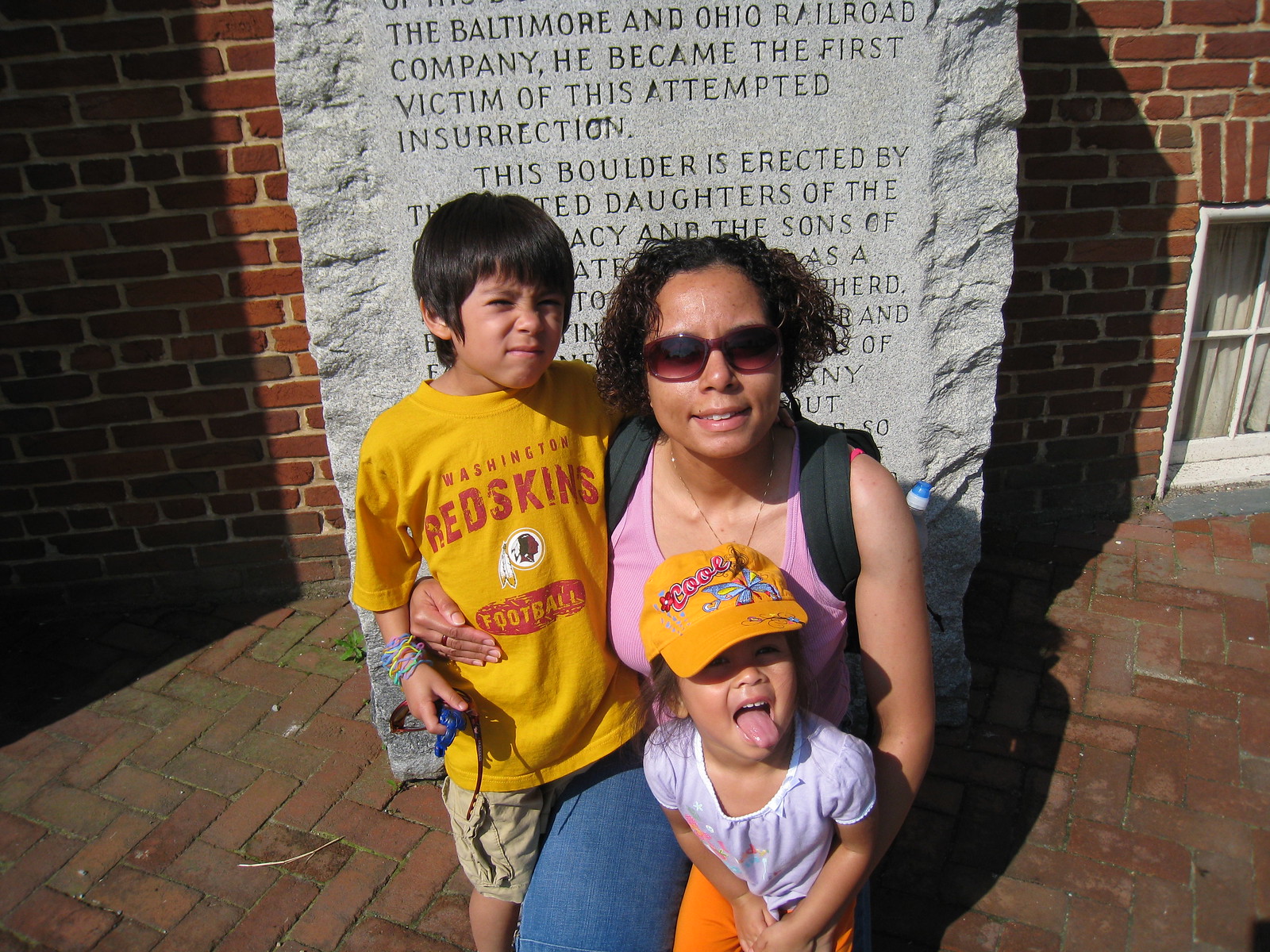This is a color photograph taken outside on a sunny day, capturing a tender family moment. A woman with short, curly brown hair, wearing sunglasses, a pink tank top, blue jeans, and a backpack, is kneeling on a brick sidewalk. She is embracing two children: a young boy and a younger girl. The boy, standing to her right, has his arm around her and she reciprocates by wrapping her arm around his waist. He has short black hair and is dressed in a yellow Washington Redskins football shirt. On her lap, sits a little girl, about two or three years old, dressed in a white top, orange pants, and a yellow hat. The girl playfully sticks her tongue out at the camera. Behind them is a large, chiseled stone monument with smooth sections that features engraved text. Most of the inscription is obscured by the family, but visible words include "Baltimore and Ohio Railroad Company," "He became the first victim of this attempted insurrection," and "This boulder is erected by... Daughters of the Confederacy." In the background, a brick building is partially visible, adding to the historic ambiance of the scene.